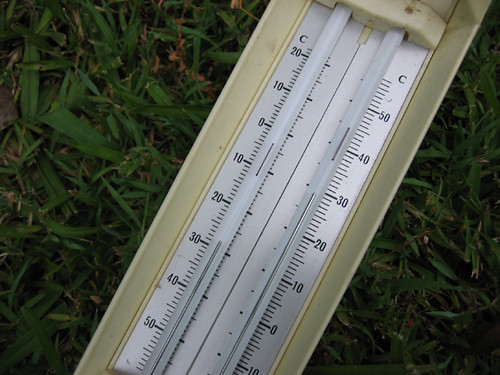A specialized bifurcated thermometer designed to record high and low temperatures since its last reset. The device features two mercury-filled tubes, both calibrated in centigrade but with different scales on each side. The left tube measures the lowest temperature, ranging from 20°C to as low as -60°C, while the right tube tracks the highest temperature, spanning from -10°C to 60°C. Each tube contains a column of mercury, which is silver in color, with an additional thin segment of mercury above the main column. This segment marks the peak or trough of the temperature recorded until the thermometer is reset by shaking. The tubes are encased in a yellow plastic frame with a white scale card for easy reading.